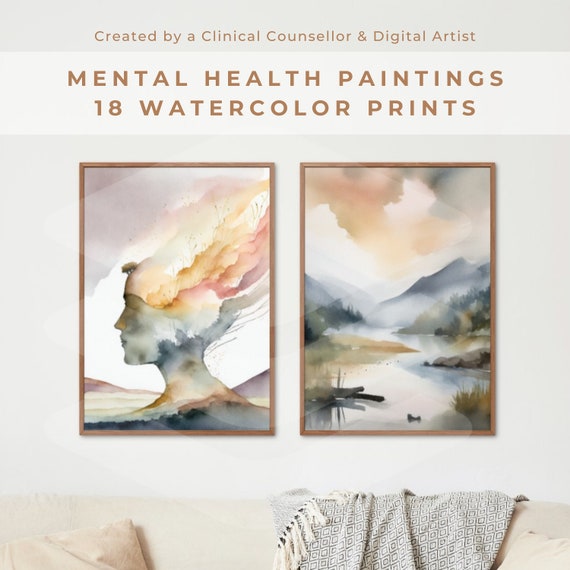This detailed image captures two stunning watercolor prints titled "Mental Health Paintings, 18 Watercolor Prints," created by a clinical counselor and digital artist. Set in portrait mode, the photo showcases these vibrant artworks mounted on a wall behind a cream-colored couch adorned with a gray throw blanket and a pillow, creating an inviting atmosphere.

The first painting features a side profile of a woman whose hair, colored in an array of rainbow hues, seems to be blowing upwards, merging with the sky. Her face is painted primarily in blues, with darker blue shadowing at the back of her head and some tan tinges on her neck, set against a backdrop of white and what appears to be a hill.

The second painting portrays a serene water scene with a duck floating on a stream that winds between patches of land, leading towards mountains and a brilliantly colorful sky filled with hues of yellow, red, and tan. Both images combine to form a harmonious and serene setup, illustrating the creative fusion of mental health themes conveyed through watercolor art. The text at the top of the image, in rust-colored font, references the artist's dual expertise and the series of 18 prints.